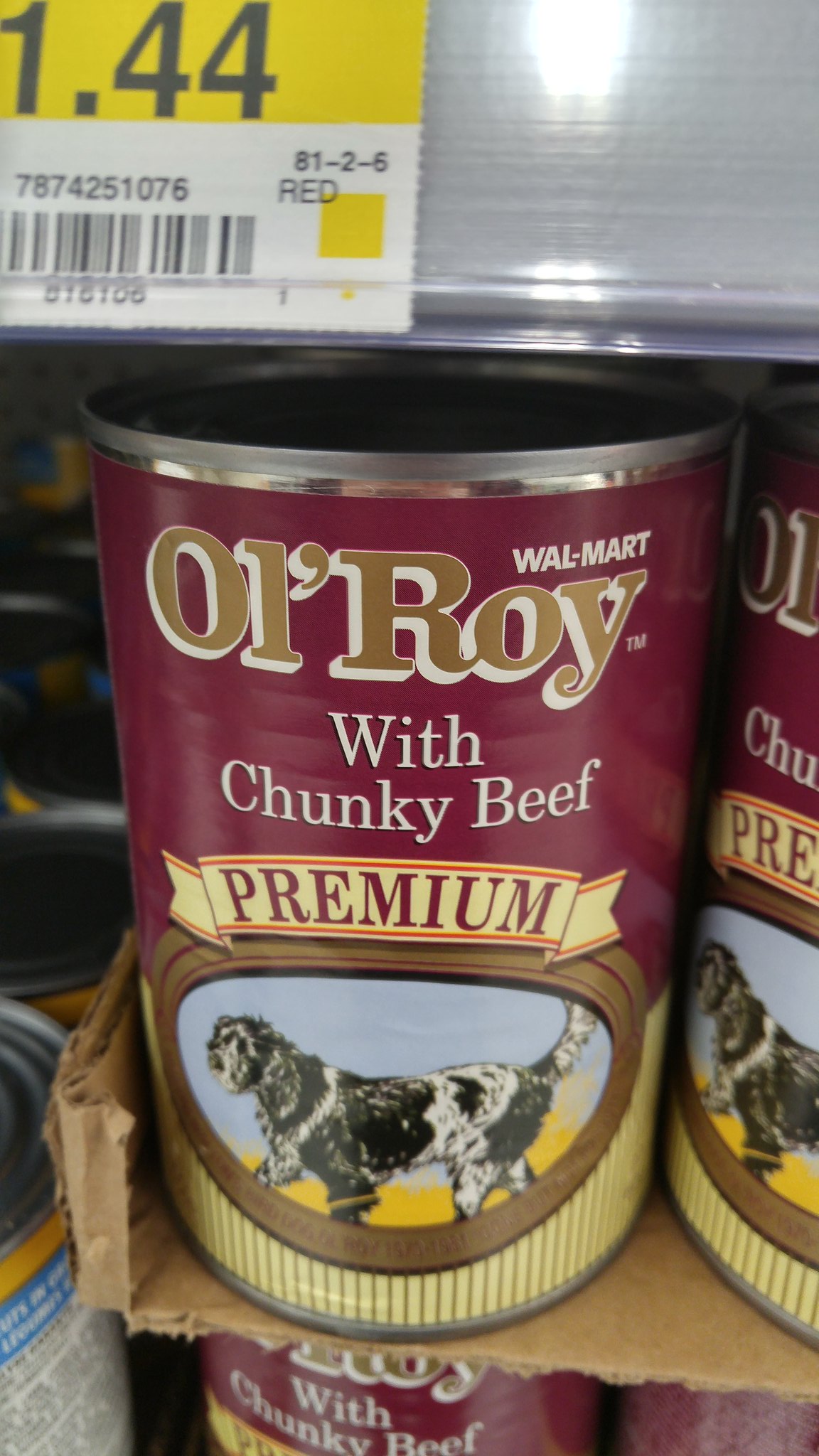The image captures an old, maroon can of Ol' Roy Chunky Beef Premium dog food located on a Walmart store shelf. The can prominently features a vintage Walmart logo and a detailed label, predominantly maroon with a circular blue and yellow background showcasing a black and white dog. The label's intricate design includes the brand name "Ol' Roy" in brown, "Chunky Beef" in white text, and "Premium" in red text on a yellow banner. Above the can, a price tag is visible, reading $1.44 on a yellow background. The image also shows the can stacked among others of the same type, indicating a store setting.